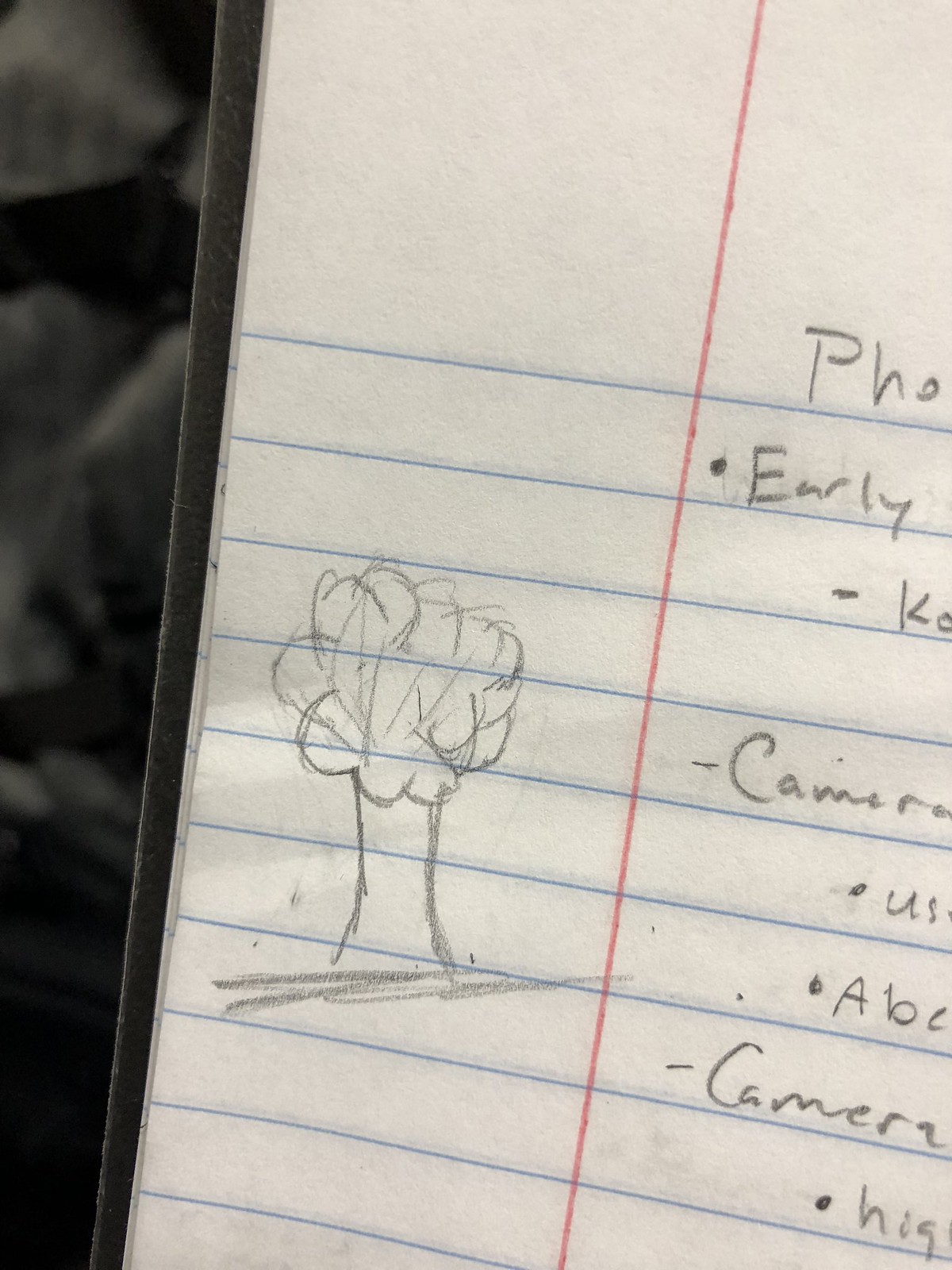The image depicts a close-up of a partial piece of wide-ruled notebook paper with blue horizontal lines and a distinctive red vertical margin line. Dominating the left side of the paper is a simple pencil drawing of a tree, featuring a thick trunk and a scalloped, leaf-laden treetop, shaded for texture, with horizontal lines below suggesting ground. On the right side of the frame, the top portion shows the start of some handwritten notes in pencil, though many words are cut off. Legible text includes "early," "ko," and "camera," with additional bullet points listing "use," "a b e," and "hi," although these are also partially obscured. In the blurred left margin area, a small black spot is visible, suggesting either a shadow or off-frame object.